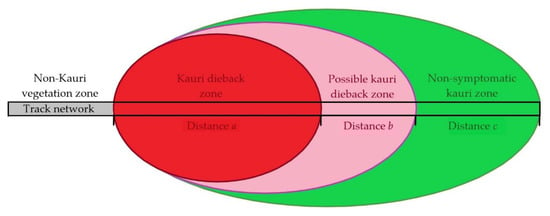The image is a detailed educational or instructional diagram displayed on a white background. It features three nested ovals: a large green oval, a medium pink oval inside the green one, and a smaller red oval nested within the pink one. The green oval is labeled "non-symptomatic cowrie zone distance C," the pink oval is labeled "possible cowrie dieback zone distance B," and the red oval is labeled "cowrie dieback zone distance A." A black, slender rectangular line runs horizontally through the center of the ovals. To the left of the ovals, the diagram includes the label "non-cowrie vegetation zone track network."